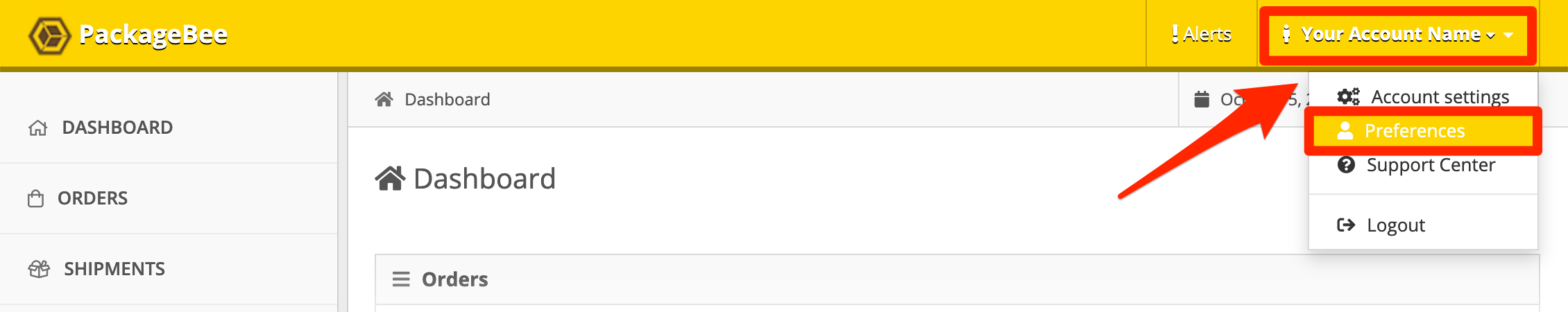This screen capture features a user interface with a gold bar at the top, displaying "Package B" in white font alongside a black, square logo with a gray cube inside it. To the right, "Alerts" is written in white font with an accompanying exclamation mark. 

Below this, the account name is highlighted with a red box, a white pull-down menu, and a small person icon next to it. A red arrow points upwards towards the account name.

Further down, a sub-menu on a white background is revealed. The options include "Account Settings" with a cogwheel icon, "Preferences" highlighted in yellow with a person icon, "Support Center" with a question mark icon, and "Logout" with a box and an arrow icon.

To the left, the menu has a gray border. It lists "Dashboard" with a home icon and a cut-off date featuring a calendar icon. Other options include another "Dashboard" and "Orders" with three lines, although the rest of this left menu is obscured.

On the right side, below "Package B," the options "Dashboard" with a home icon, "Orders" with a shopping bag icon, and "Shipments" with a gift box icon are visible.